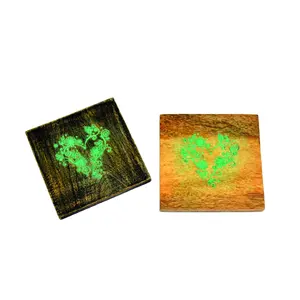In the image, there are two square-shaped objects side by side against a plain white background, each possibly serving as coasters or decorative tiles. The object on the left is characterized by a dark brown, wood-like surface with visible grain patterns, and at its center is a heart-shaped design made of vibrant green vines, giving a glowing or highlighted effect. The object on the right contrasts with a lighter, golden-brown surface exhibiting subtle variations in color from dark to light brown. Similarly, it features a heart-shaped design made of green vines at its center. The two coasters are small, each approximately three-quarters of an inch squared on screen, and are meticulously decorated with these intricate, neon-green vine hearts that add a touch of decorative elegance. The lack of text or numbers ensures that the focus remains purely on their design and texture.